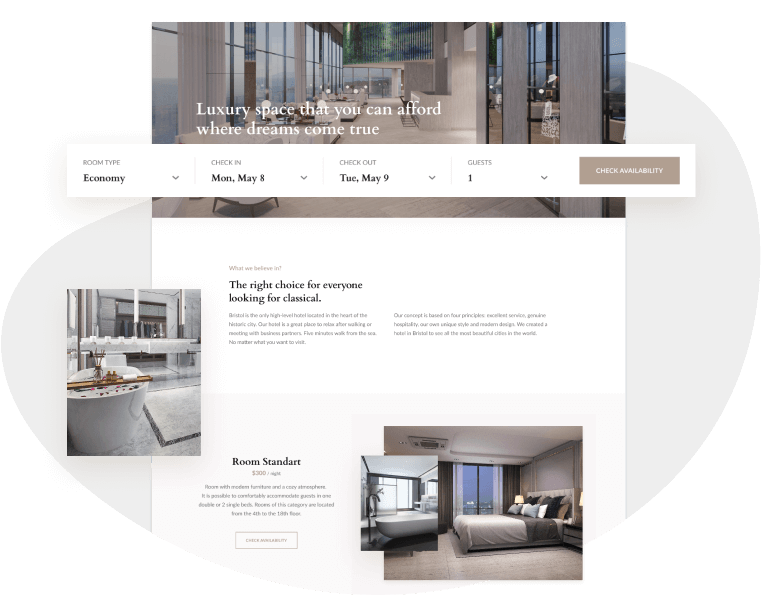The image depicts a slightly wider-than-tall website with a seamless white background. The top third showcases a banner featuring the interior of a luxurious dining hall. On the left side of the banner, there are strikingly tall windows, extending beyond a single story, suggesting extraordinarily high ceilings. Aligned below these windows are numerous dining tables adorned with white tablecloths and neatly arranged chairs, reinforcing the impression of an upscale dining area. On the right side of the banner, passages lead into additional parts of the venue.

Superimposed in the center of the banner is a message in elegant white text: "Luxury space that you can afford where dreams come true." Beneath the banner, a horizontal white bar presents various selection options: 

- Room type: Economy
- Check-in date: Monday, May 8th
- Check-out date: Tuesday, May 9th
- Number of guests: 1

To the right of this selection bar is a tan-colored button labeled "Check Availability."